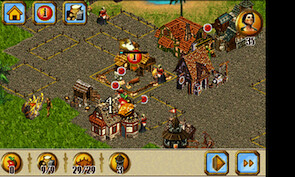The image is a detailed screenshot from a simulation video game focused on building and farming. The scene showcases a bustling, rectangular landscape with a mixture of dirt plots and greenery. The center is largely composed of parcelled farmland, interspersed with a few small buildings, including a distinctive two-story house near the center-right and a larger building behind it. To the lower-left are three more structures, one that resembles a house and another that could be a barn. The terrain is slightly angled, giving the plots a tilted appearance.

In the top part of the image, a water source is visible, while green grassy areas flank the left side. Small, indistinct figures, possibly the game's inhabitants, can be seen moving about, marked by red dots likely used for interaction. 

Overlaying the gameplay area, a circular avatar of a man's head and shoulders is situated in the upper right. Adjacent to this are three blue-background icons: a house, an informational 'i', and an indistinguishable third icon. The bottom of the image features a control bar with four yellow-gold circles, each showing different quantities, and more blue-background squares. Among these, one clearly contains a play button and another a fast-forward button. Additionally, there are two blue squares on the bottom—one containing a single diamond-shaped object, the other containing two. This comprehensive setup suggests a play area where players strategize to build, farm, and manage resources.